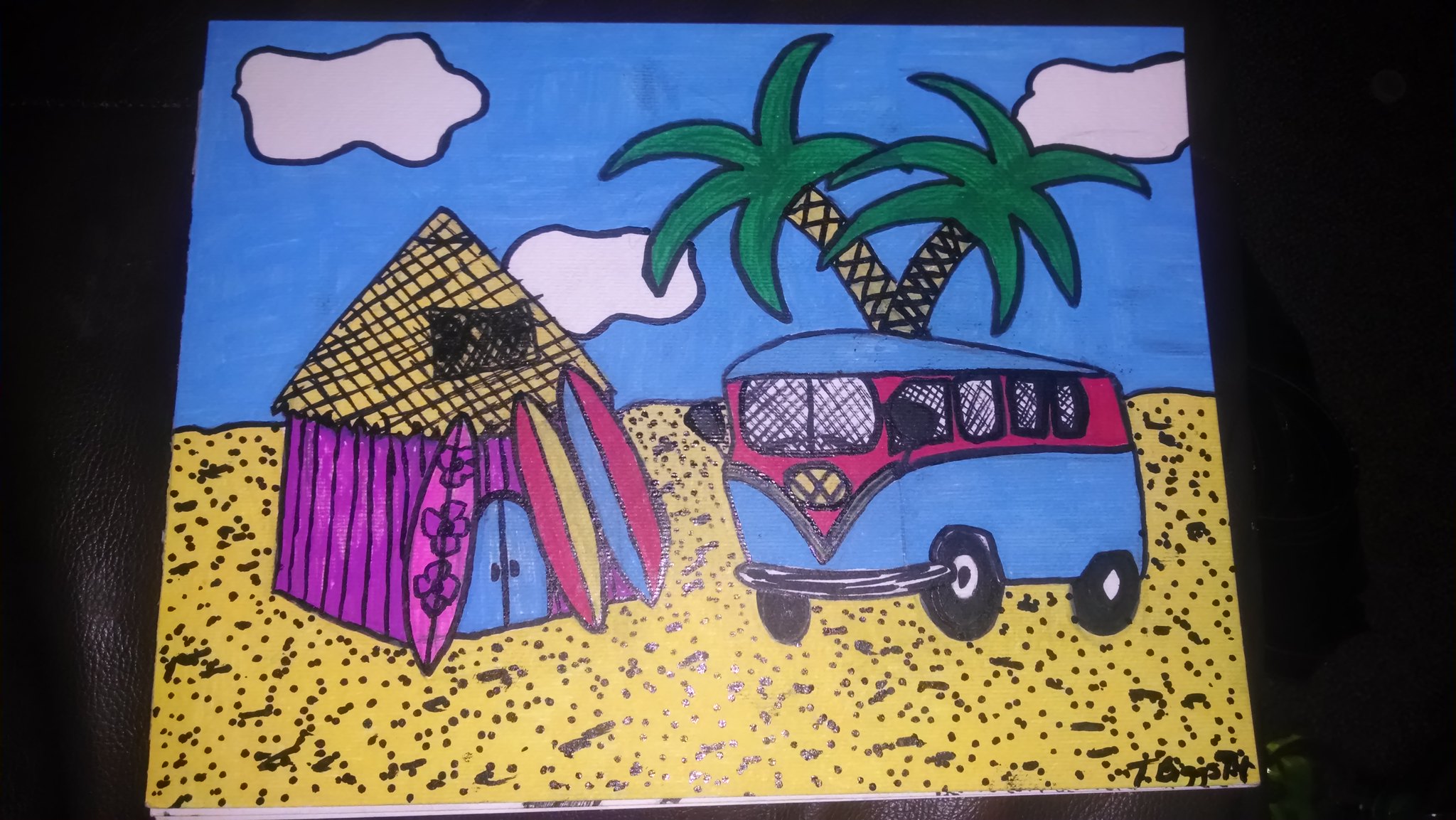This image captures a detailed sketch on a black fabric surface. The vibrant marker drawing depicts a serene beach scene, featuring a yellow sandy shore. Prominent in the sketch are two palm trees with distinctive yellow trunks and lush green leaves, standing majestically against a bright blue sky dotted with fluffy white clouds. To the side, a quaint purple shack with a yellow straw roof adds to the tropical ambiance. Leaning against the shack are several surfboards, including a notable purple one adorned with purple flowers. Additionally, a blue bus with striking red detailing is parked nearby, prominently displaying a golden Volkswagen logo encircled on the front. The artwork is rich in color and detail, evoking a lively and welcoming coastal atmosphere.